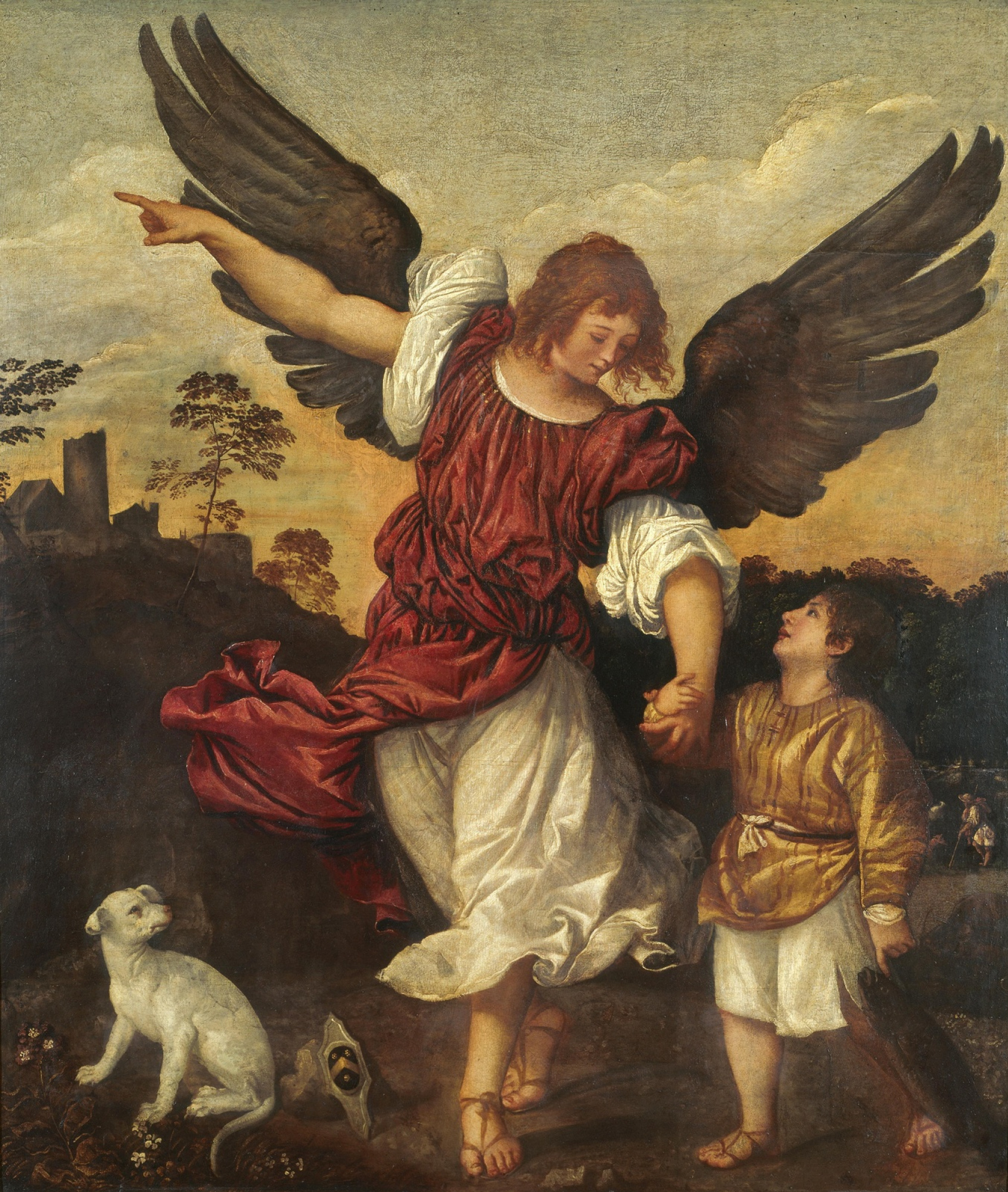This captivating pre-Raphaelite oil painting, vertically oriented, depicts an ethereal outdoor scene. At the center is a red-haired angel with dark, possibly black, wings. She wears a flowing white robe adorned with a smaller, burgundy-red robe, and strappy sandals. Her red curly hair cascades to her shoulders as she points off to the left, guiding the viewer's gaze. Besides her, walking hand-in-hand is a small boy, seemingly around six to eight years old, with brown hair and clad in a gold tunic over a white robe, also wearing strappy sandals. In his left hand, he holds an indistinct object. The angel's downward glance and the boy’s upward gaze create a nurturing dynamic between them. At the bottom left, a small white dog looks up at the pair with attentive eyes.

Behind this celestial duo, the landscape showcases muted natural tones, with dark trees and a possible farm building in the distance. The sky above is a moody medium blue, interspersed with white clouds and tinges of red, perhaps suggesting a sunset. The entire composition is suffused with an air of otherworldly tranquility and timelessness.